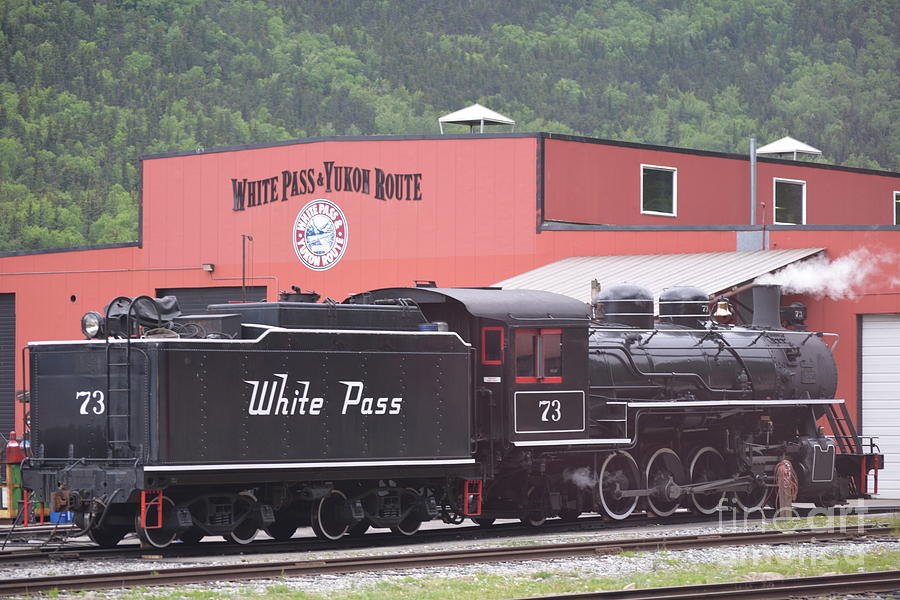This color photograph, taken during the daytime, captures a steam locomotive, prominently positioned in the center with a three-quarter view from the rear. The inactive, yet steaming black locomotive, marked with the number 73 and "White Pass" on its tender, showcases a 2-8-2 narrow gauge wheel arrangement. Directly behind it stands a modern, orange building adorned with "White Pass and Yukon Route" in black lettering and a distinct large circular symbol below the name. Beyond this structure, a lush, green hillside densely covered with evergreen trees stretches upwards, creating a scenic backdrop. Train tracks run along the bottom of the image, grounding the locomotive in its station setting, while the vibrant train and station building dominate the central frame, juxtaposed against the natural beauty of the hillside.